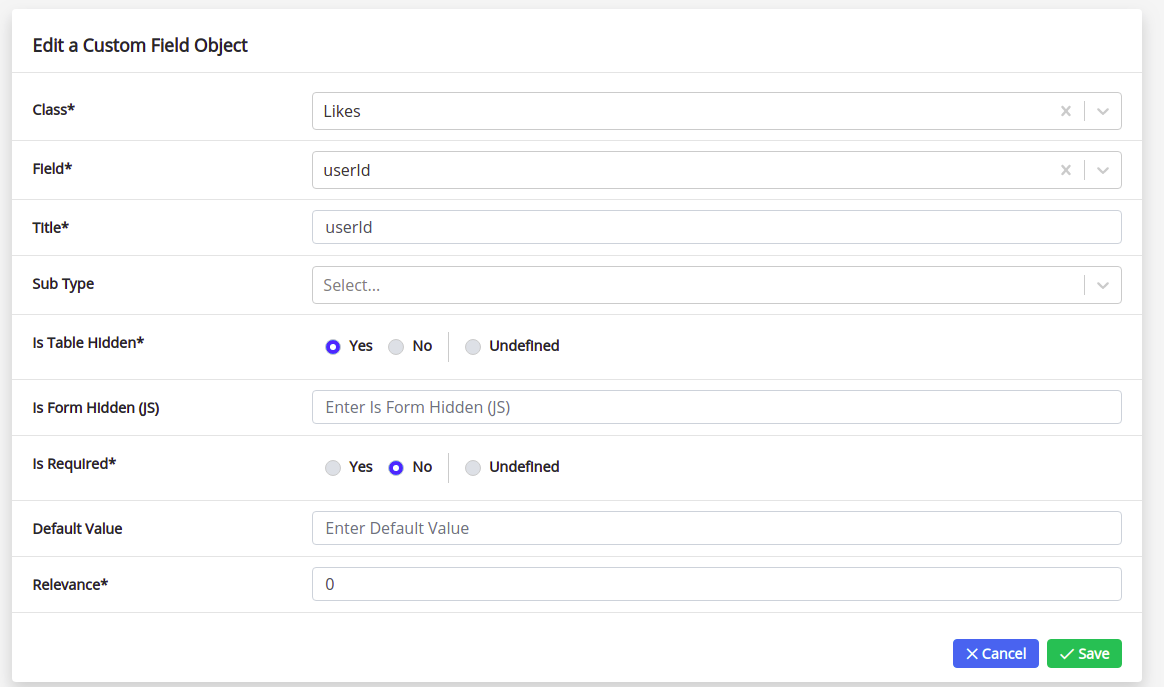This screenshot captures a form interface with various options displayed on a light gray background, overlaid by a central white rectangle. At the top left of the rectangle, the bold black text reads "Edit a Custom Field Object." The form is divided into distinct sections by thin gray lines running horizontally across the white rectangle, neatly organizing the interface.

### Detailed Breakdown:

1. **Class***: The title on the left side is in bold black text, adjacent to a dropdown menu displaying "Likes."
2. **Field***: Another bold black title on the left, with a dropdown menu set to "User ID."
3. **Title***: Repetition of the same layout - bold black title with the dropdown menu also set to "User ID."
4. **Sub Type**: Accompanied by a dropdown menu that shows "Select..." in light gray placeholder text.
5. **Is table hidden***: This section features three radio buttons:
   - "Yes" (selected with a blue donut indicator)
   - "No"
   - "Undefined" (separated from the others by a thin vertical gray line)
6. **Is form hidden (JS)**: Next to this text is a textbox with light gray placeholder text reading "Enter is form hidden (JS)."
7. **Is required***: This section mimics the radio button layout of "Is table hidden," but here "No" is selected with a blue donut indicator.
8. **Default value**: This field is simply listed without additional input options.
9. **Relevance***: Concludes with a similar presentation - bold black title on the left side.

Every field title employs bold black text for clarity, with dropdown menus, text boxes, and radio buttons providing interaction points for the user. The interface design ensures that each section is distinctly separated, aiding in user navigation.